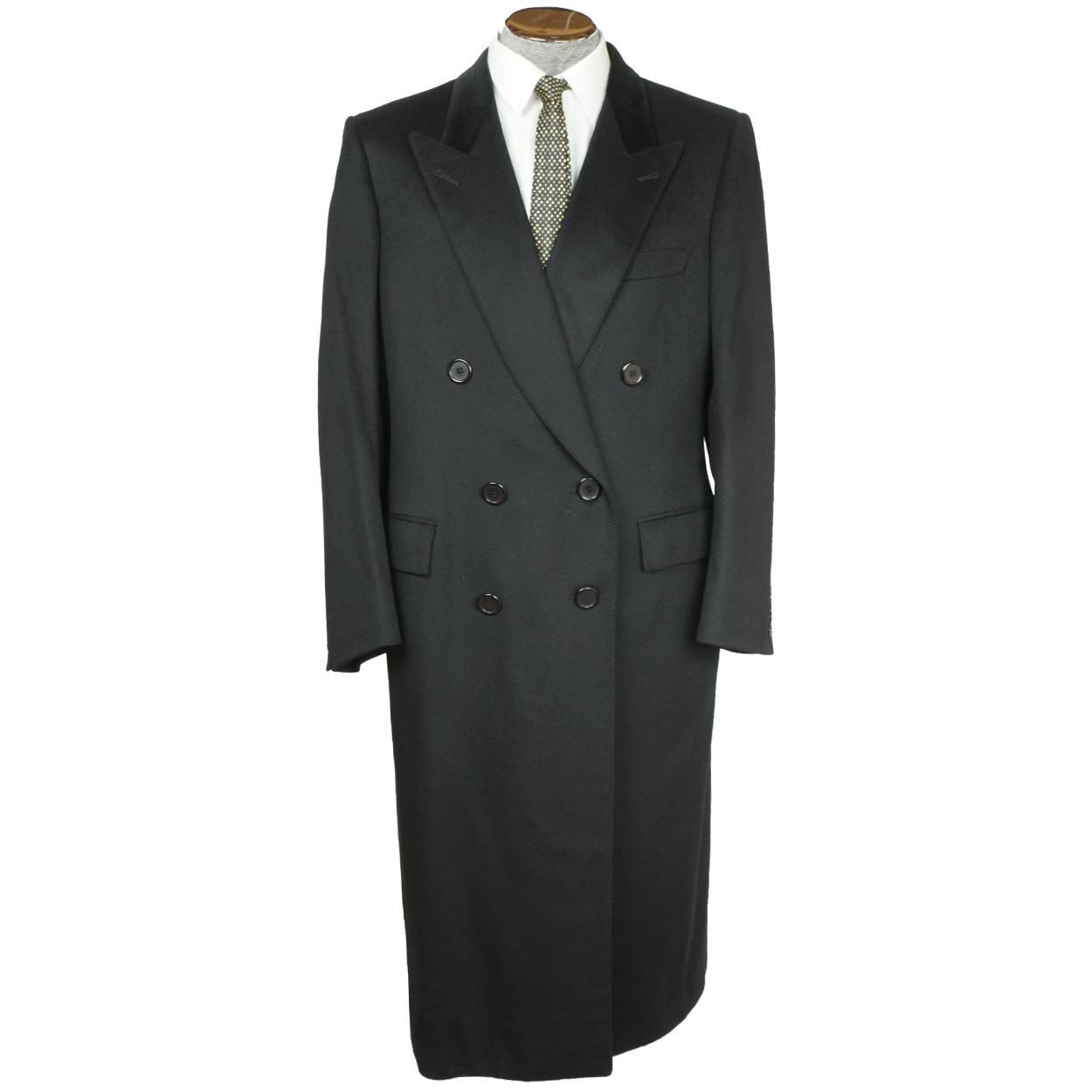The image depicts a long trench coat, appearing to be either dark blue or black, draped over a headless, wooden mannequin. The background is a clean, well-lit white, giving the image a minimalistic and sterile look. The trench coat is notably lengthy, potentially extending down to the knees or ankles, and features six buttons on the front along with two pockets, one on each side. Underneath the coat is a white button-up shirt paired with a black and white dotted tie. The neck area of the wooden mannequin is visible, resembling a flat, circular piece of wood, adding to the simplicity and focus on the garment itself.